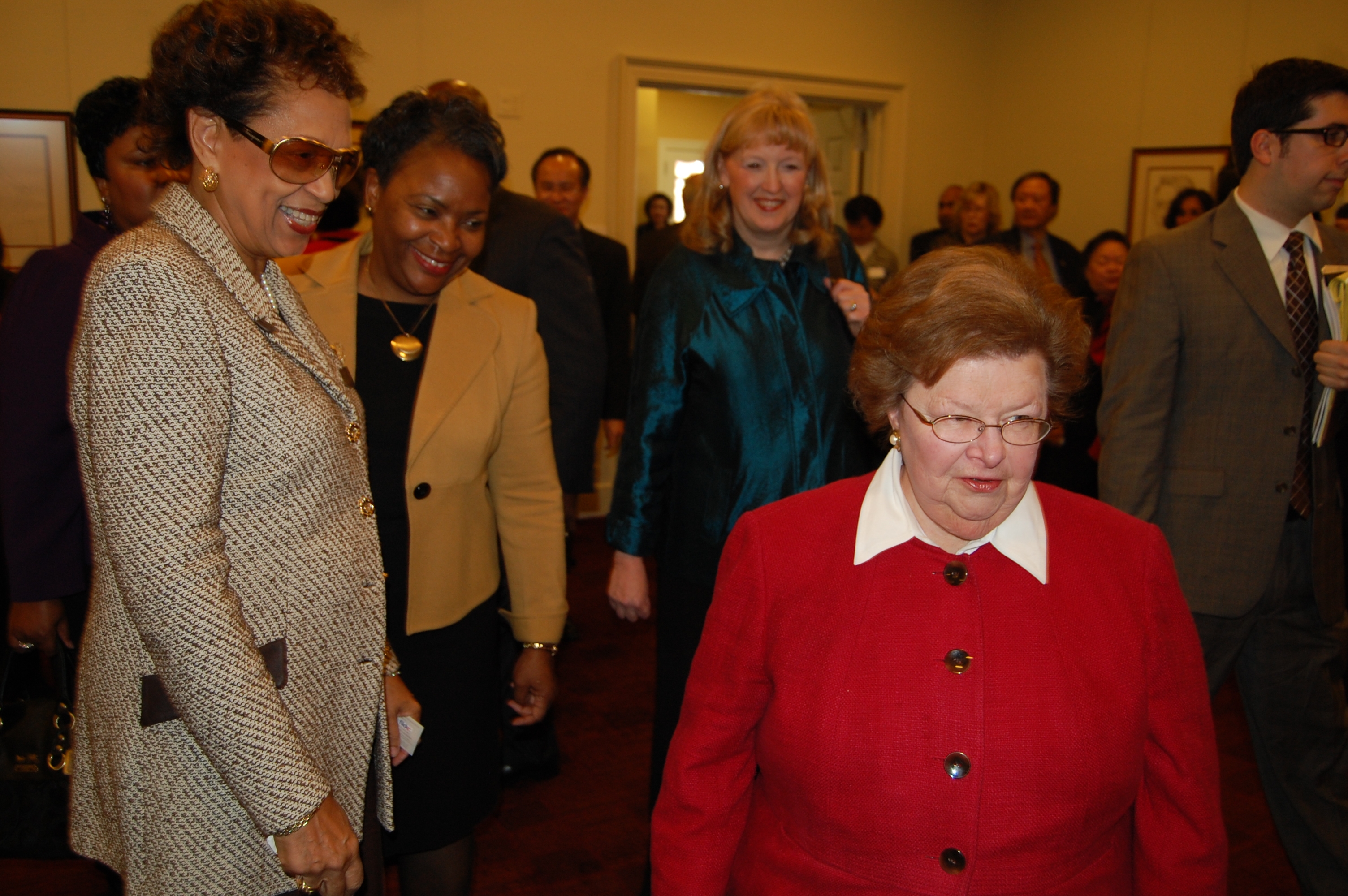The image captures a bustling indoor event, likely a formal gathering or business meeting, with around 20 well-dressed attendees. Predominantly attired in business or church-style clothing, the participants' attire includes suits, blazers, and dress tops. 

In the foreground, an elderly, slightly heavy-set Caucasian woman with short dyed-red hair and thin wire glasses is prominent. She dons a red suit jacket with a white collared undershirt, fastened with four visible black buttons. This woman's gaze is directed towards the lower right corner of the image.

To her left, a medium-toned black woman stands, her hair elegantly styled up and adorned with large dark glasses. She is dressed in a tweed suit jacket and similarly looks towards the same direction as the elderly woman.

Other visible attendees include a younger woman in a teal outfit and another black woman, along with additional individuals in the background. The backdrop features light yellow or white walls, likely altered by lighting, adorned with pictures that are partially obscured. 

A man in a business suit—with glasses and holding an object against his chest—is also noted on the right side of the image. The overall direction of everyone's gaze suggests they are collectively examining something, potentially indicative of a focal point such as a presentation or display.